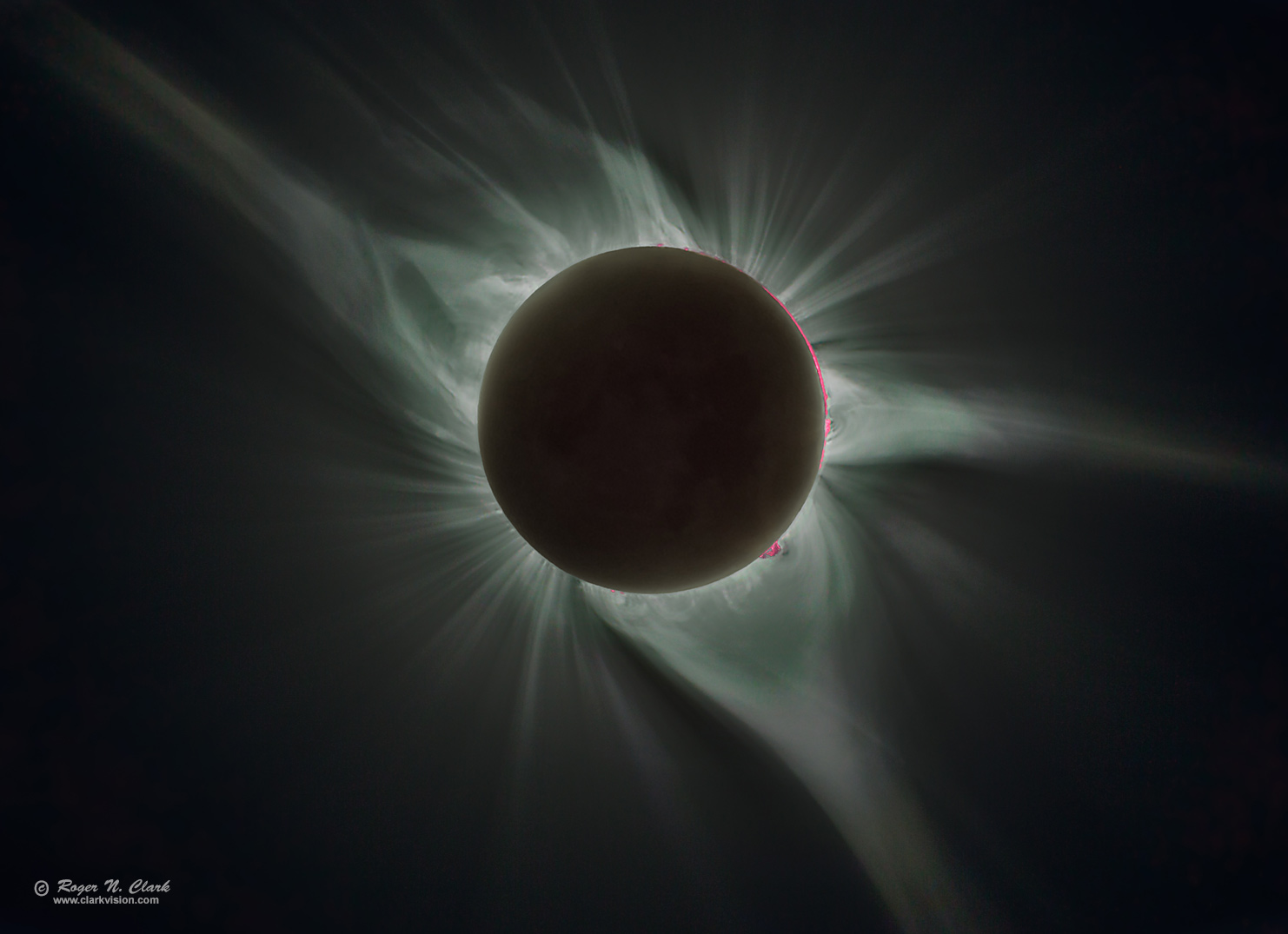A striking, AI-generated photograph capturing the moment of totality during a solar eclipse, featuring a predominantly black and white palette with subtle pink accents along the edges. At the center, a dark disc, presumably the moon, obscures the sun, giving rise to ethereal, gray-toned streams of light that stretch outward into the charcoal-gray sky. This captivating image, marked by a hint of red on the moon’s edge, emphasizes the contrast between the darkened sky and the delicate flares of sunlight. The photograph, labeled with the name Roger N. Clark and the website www.clarkvision.com at the bottom left, creates a dramatic and surreal visual that underscores the ephemeral beauty of astronomical events.